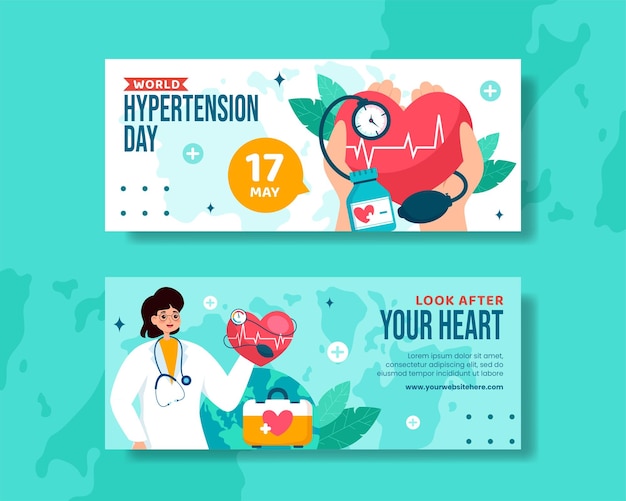The image features a vibrant, informative design centered on promoting World Hypertension Day, set against a seafoam green background with darker teal decorative elements resembling a world map. At the top, a white rectangular banner prominently displays "World Hypertension Day" in bold red and blue letters. Below the text, a gold circular emblem with "17" at the top and "May" at the bottom highlights the date of the event. 

In the upper section of the image, a large, stylized heart takes center stage, complete with a zigzag white line and an attached black pump used for measuring blood pressure. The heart is flanked by green leaves, with a circular gauge wrapping around the background. A blue medicine bottle with a heart sticker and cap is situated just beneath the heart.

The lower section features a teal rectangle showcasing a female doctor dressed in a white lab coat, yellow shirt, and glasses, holding a heart similar to the one above. The heart in her hand also includes a stethoscope and blood pressure gauge. Adjacent to her is a yellow cooler with a white top, bearing a heart symbol and surrounded by multiple plus signs. 

Overlaying the world map design in the background, bold red text at the top reads "LOOK AFTER," and large blue letters state "YOUR HEART." Below this message, there is a paragraph of detailed information and a website link in small, dark blue font. This compelling composition effectively conveys the importance of heart health and awareness of hypertension.